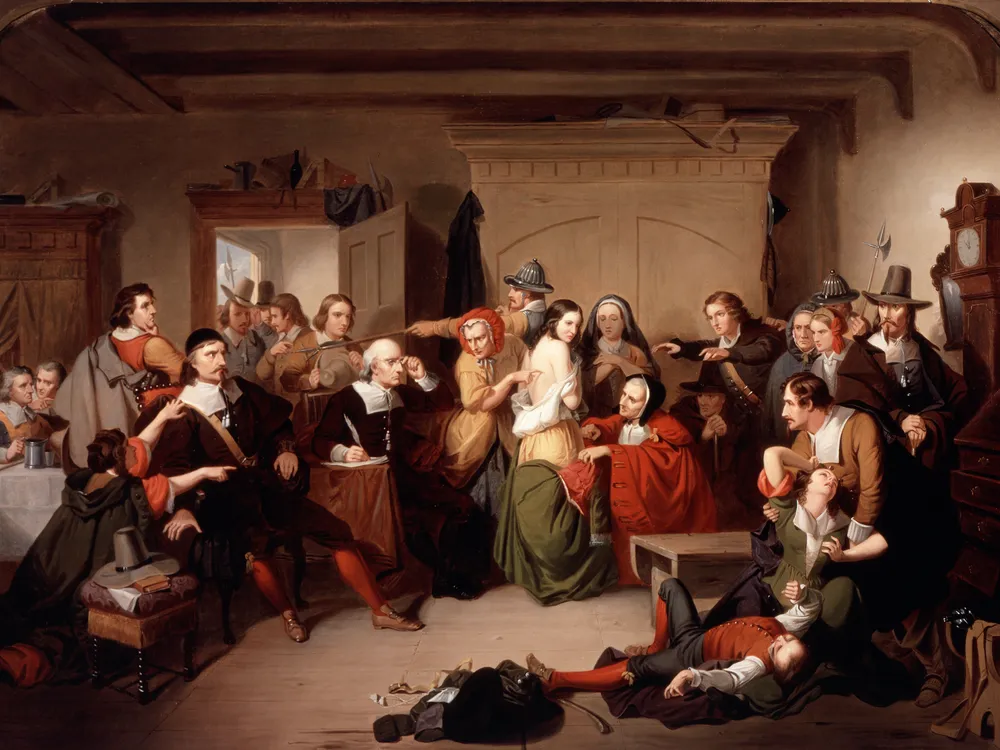This captivating painting, likely dating from the 1600s to 1800s, depicts a crowded and chaotic scene, set in what could be a museum-worthy framed piece. The room is teeming with approximately 30 individuals, adorned in period-specific attire, including voluminous dresses that envelop the wearers and old-style helmets and hats. The atmosphere is tense, with soldiers, distinguishable by their presence and possession of axes, rather than guns, directing the commotion.

Central to the scene, a dramatic event unfolds: a man on the ground and another man cradling a woman who appears to have just collapsed, with lifeless bodies dotting the chaotic scene. Amid this turmoil, a figure brandishes a stick or spear menacingly at a seated individual, drawing the attention of almost everyone around. Fingers are pointed in various directions, as onlookers concentrate primarily on the man in the chair. The room itself contains a large wardrobe and an open door leading to another space, enhancing the sense of depth and disorder.